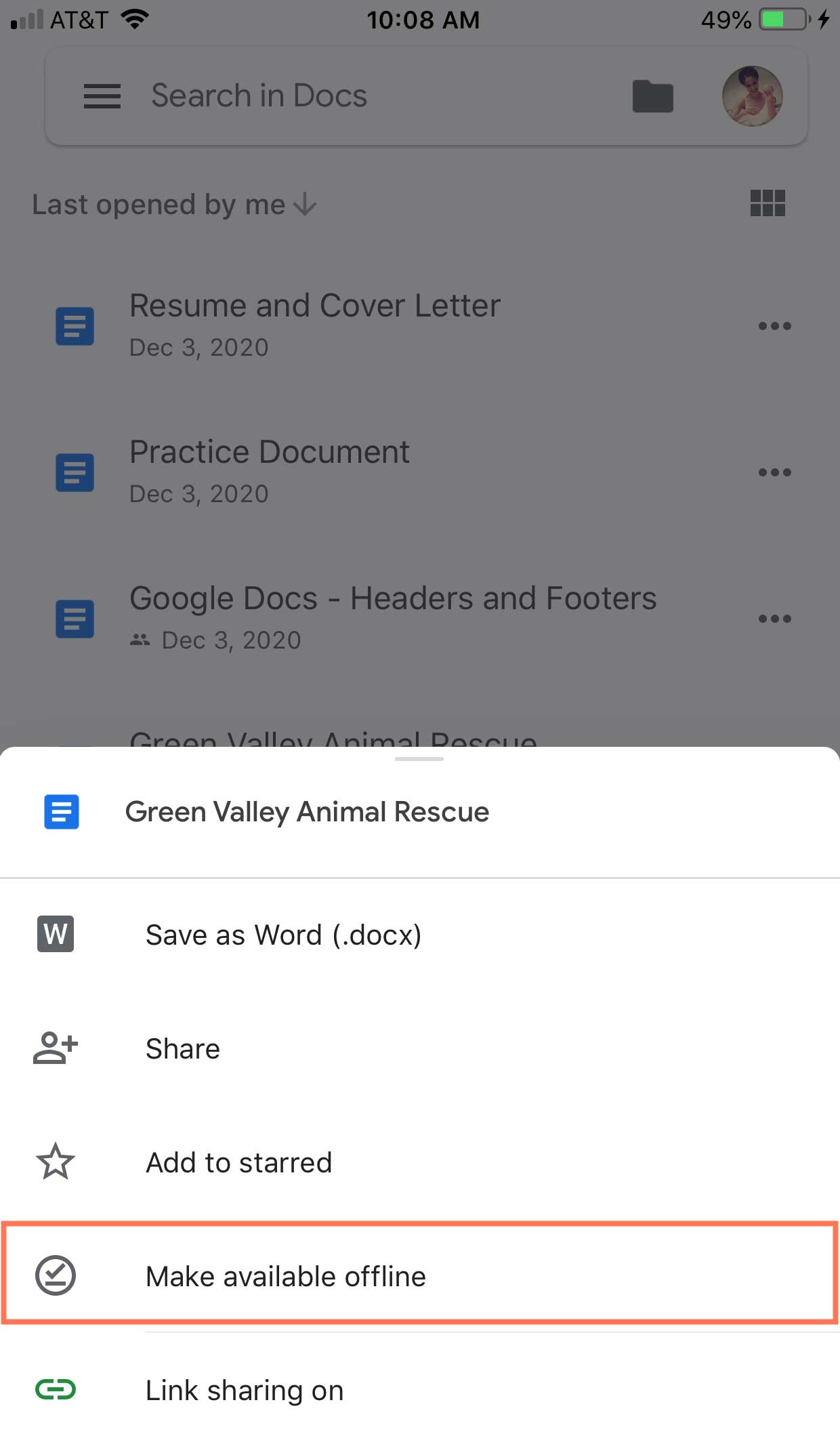This image displays a computer's cell phone screen with a detailed view of its interface. The upper section of the screen is entirely gray, while the bottom section is white, indicating a dual-toned layout. At the top, there are several options: "Search in docs," "Resume and cover letter," "Practice document," and "Google Docs - Headers and footers." Some listed dates include December 3rd, 2020, which appears to be when these documents were created.

Moving down, the first section is labeled "Green Valley Animal Rescue," separated by a faint gray line from the next section. This subsequent section is labeled "Save as Word Docs," featuring a boxed W symbol. Below this, there's a clickable "Share" option accompanied by a silhouette of a person with a plus sign. Adjacent to it is the "Add to starred" option, indicated by a star icon. 

Notably, there's a rectangular area outlined in red with the text "Make available offline," alongside a circle containing a check mark. The final option displayed is "Link sharing on," symbolized by a paperclip icon. This comprehensive arrangement of options and tools suggests the image captures a Google Docs interface, providing various document management features.